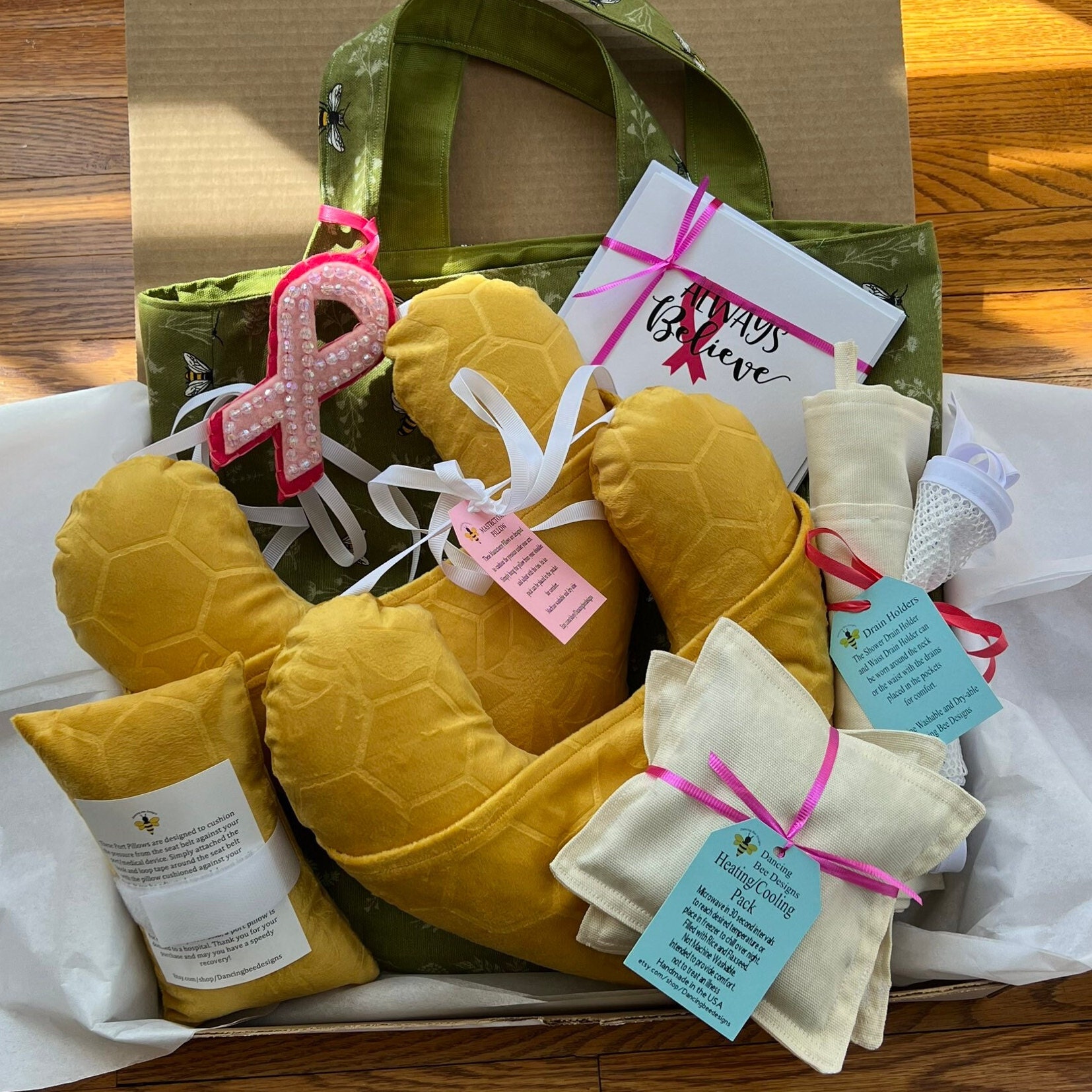In the image, we see a carefully organized care package containing a variety of comforting and thoughtful items. Dominating the foreground are two yellow neck pillows, intricately designed with a honeycomb pattern and adorned with bee icons. Alongside these is a matching small rectangular pillow. Notably, there are also off-white fabric heating and cooling packs, each wrapped neatly with a bright pink bow and labeled with a blue tag that reads "Dancing Bee Designs Heating/Cooling Pack", with some fine print indicating they are handmade in the USA.

There is also a visually striking pink ribbon icon, typically associated with breast cancer awareness, fashioned in a stuffed-animal style for added charm. A notebook prominently displays the inspirational message "Always Believe". Behind it, a purse decorated with bee designs is visible, enhancing the thematic coherence of the package.

Additionally, the package includes linen squares, possibly napkins or hand towels, tied up with ribbons for a neatly-presented appearance. A green shopping bag with cloth handles can be seen, decorated with a dangling ribbon. All items are set against a backdrop of white tissue paper, all housed within a box, creating an organized and inviting presentation.